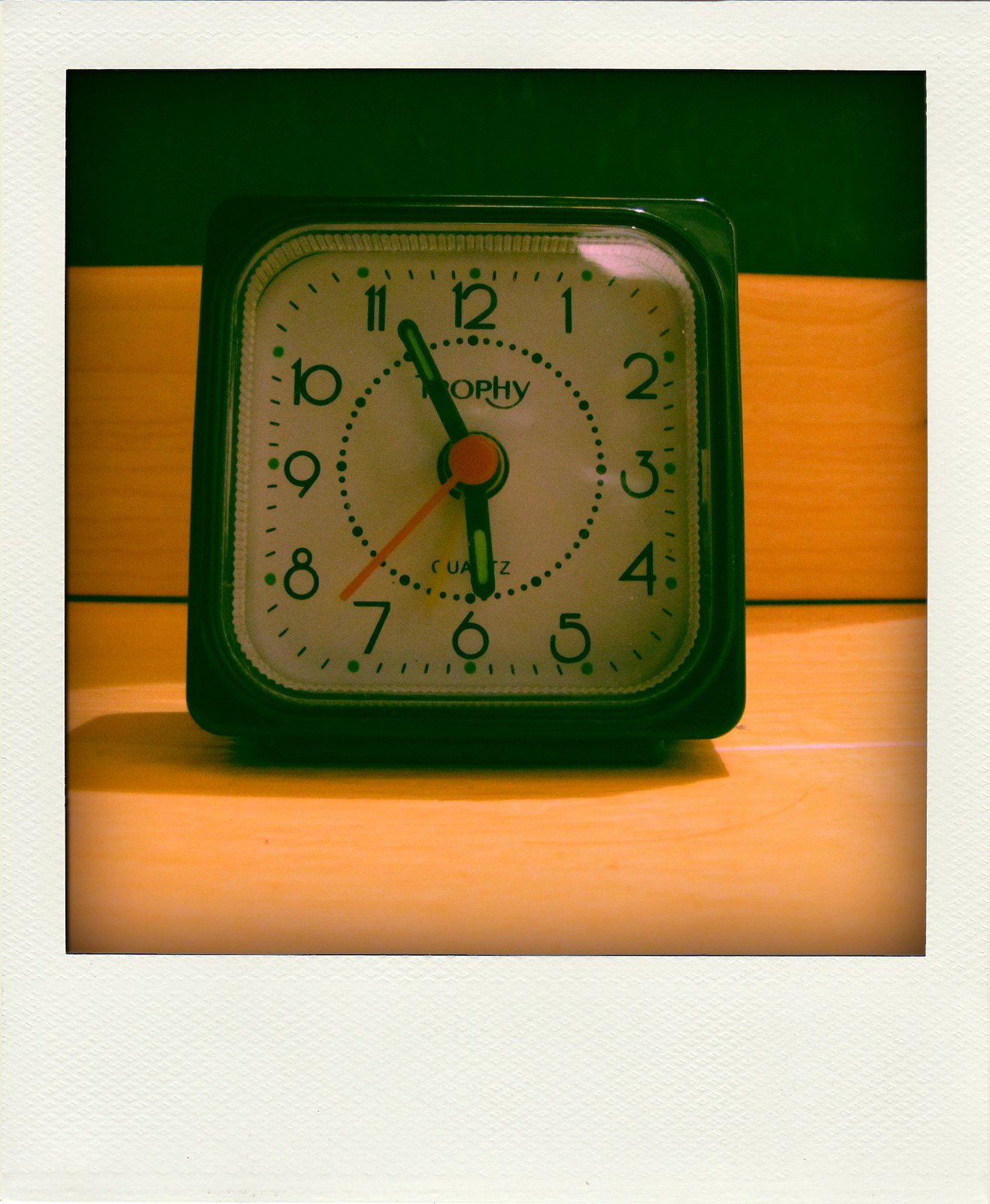This image features a small, square-shaped alarm clock made by Trophy, branded with the name "Trophy Courts." The clock is predominantly green with matching green digits and hands, accompanied by a vibrant red second hand. It displays the time as 5:55. A clear glass cover protects the clock face. The clock is set against a wooden surface that complements the green-painted wall in the background. The design includes an inner square frame around the white clock face, adding a crisp contrast to the overall aesthetic.